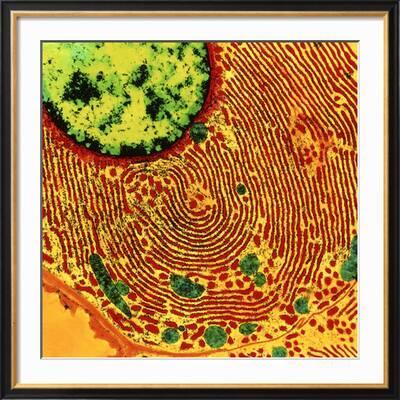The photograph captures a richly framed piece of contemporary art. The frame itself is an elegant combination of black and gold, complemented by a pristine white matte. The artwork is set against a bold, yellow painted background, where the focal point features a striking motif reminiscent of a thumbprint or fingerprint. Radiating from the center are dynamic red lines that intermingle with the yellow, creating a sense of movement and depth. The vibrant composition is accentuated with touches of green; most notably, a fluorescent lime green circle, marked with darker patches, intrudes from the upper left, adding a contrasting element. Additionally, small green dots punctuate the lower portion of the painting, contributing to the overall lively and textured appearance.